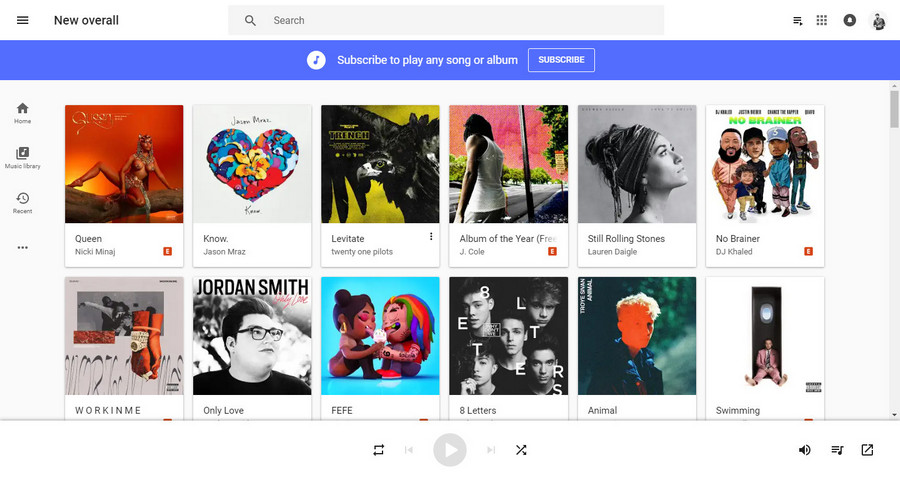The landing page of this music store or streaming service offers an inviting interface, though its name is notably absent. At the top of the page, there's a prominent search bar, which sits above a banner prompting users to "subscribe to play any song or album," accompanied by a subscription button.

Directly below this banner, there's a display of six albums in the first row, complete with album covers, titles, and artist names. The lineup includes "Queen" by Nicki Minaj, "Yes" by Jason Mraz, "Levitating" by Twenty One Pilots, "Album of the Year" by J. Cole, "Still Rolling Stones" by Lauren Daigle, and "No Brainer" by DJ Khaled.

Beneath this initial row, there's a partially visible second row of albums. Here, only the album titles are discernible while the artist names are obscured. These albums include "Workin' Me," "Only Love" by Jordan Smith (as inferred from the album art), "Effie" by Fifi Effie Effie, the song "Effie Effie", "Eight Letters," "Animal," and "Swimming."

On the left-hand side of the screen, there's a vertical navigation menu featuring icons for 'Home,' 'Music Library,' 'Recents,' and a three-dot 'Settings' option. At the bottom of the screen, there's a music player interface with essential controls: Play, Back, Forward, Shuffle, and Repeat buttons, enabling users to manage their listening experience seamlessly.